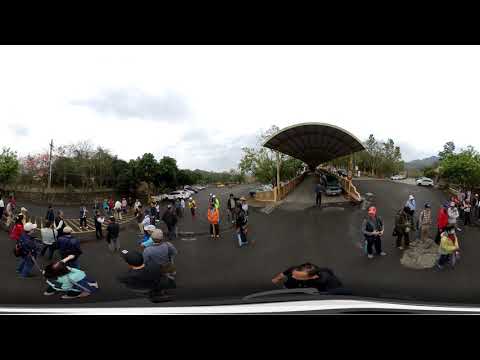The image depicts a seemingly ambiguous location that could be a bus stop, subway exit, or even a park with an unusual fan-like structure at its center, possibly serving as an awning or bridge. This structure sits above a cement driveway and emerges prominently in the middle of the panorama. Encircling this central feature, there is a parking area with cars and scattered groups of people. The surroundings include paved streets on both sides, one of which has a yellow crosswalk with people crossing. The individuals in the scene are dressed in cold weather attire such as coats and hats, suggesting an overcast day with gray, cloudy skies. The color palette of their clothing varies from grays, blues, blacks, whites, yellows, to reds. In the background, trees and additional parked cars are visible, providing a muted landscape to the overall urban setting. Due to the panoramic style of the photo, the people's bodies and faces appear distorted, adding a unique and somewhat surreal quality to the scene.